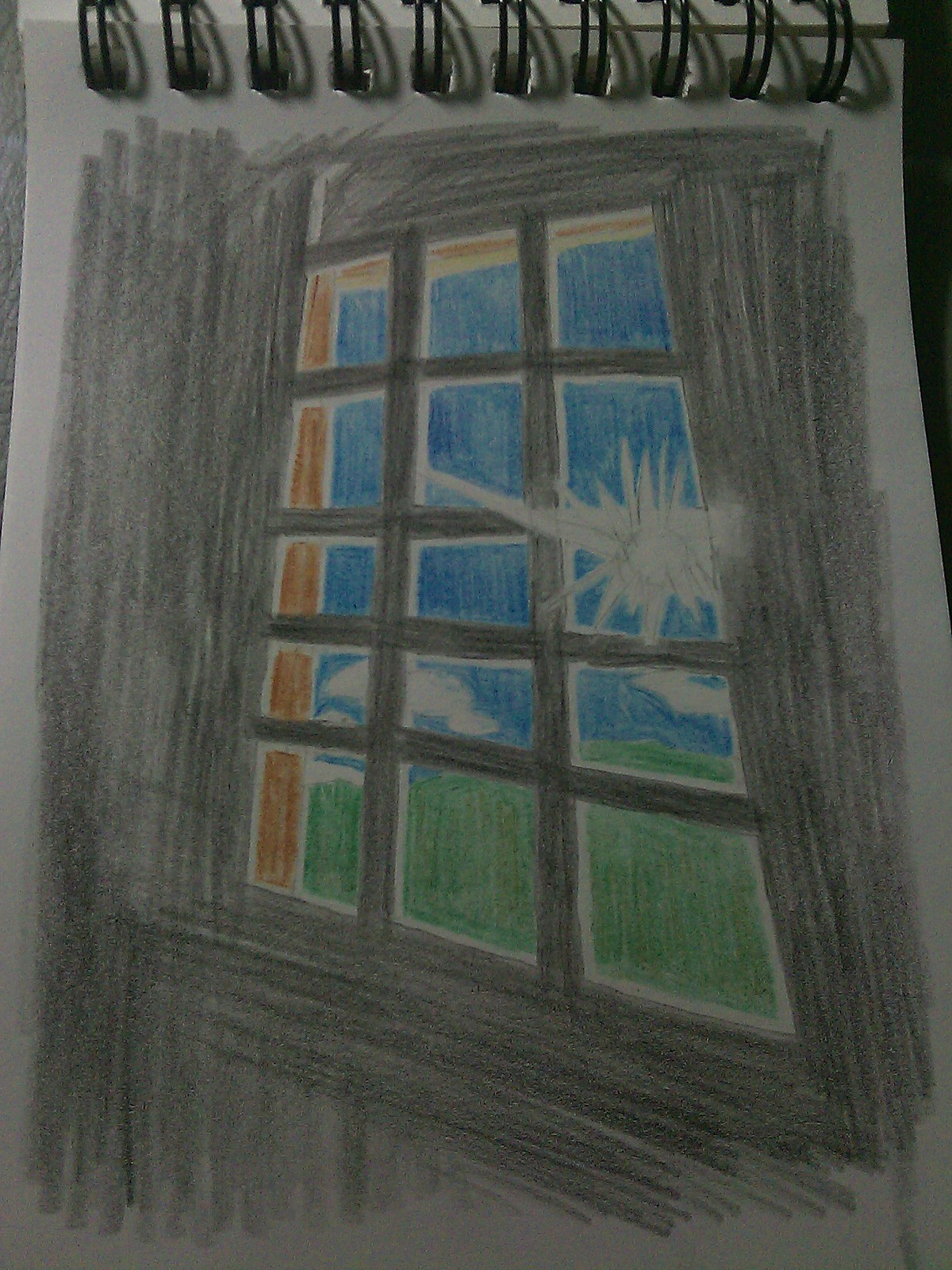This photograph showcases a vividly colorful drawing on a white notepad, secured with a black spiral ring binding. The central focus is a detailed depiction of a window with a 3-dimensional brown frame, divided into 15 individual panes. The wall surrounding the window is illustrated in shades of gray, starkly contrasting with the vibrant scene outside. Beyond the glass panes, a serene and cheerful landscape of blue sky dotted with white clouds and lush green grass stretches out. On the right side of the window, an ambiguous bright shape, possibly a sun, ball, or flash of light, adds a burst of energy to the scene. The entire artwork appears to be masterfully crafted using colored pencils, skillfully capturing the contrast between the drab interior space and the lively, inviting world outside.